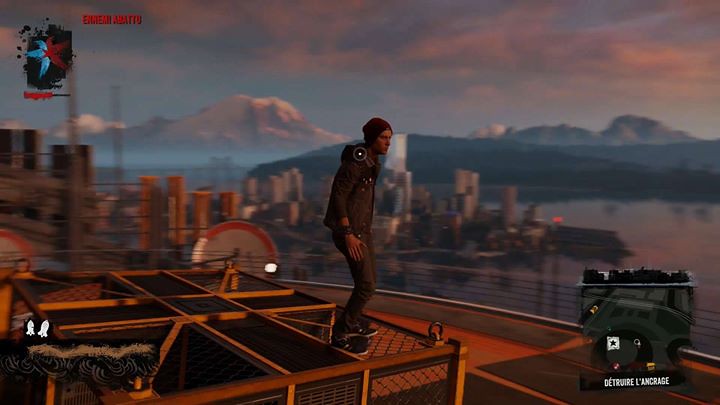This image is a still shot from the video game "Infamous Second Son" on the PS4. It showcases a third-person view of the protagonist, who wears a dark brown coat, pants, black, and white shoes, with a brown skull cap. He stands on a fence-like structure atop a rooftop, overshadowing a vast cityscape. In the distance, the city skyline features tall buildings, water bodies, and mountains with snowy peaks under a cloudy sky, hinting at a metropolitan area akin to Manhattan. The game's heads-up display (HUD) is visible, including a mini-map in the bottom right corner with French labels. Other HUD elements include a red and blue reputation bar in the top left, possibly indicating the character's morality. The bottom left corner displays two white outlined bombs symbolizing special attacks or health status, while the top right features a flower-like icon with black splattered ink around it.